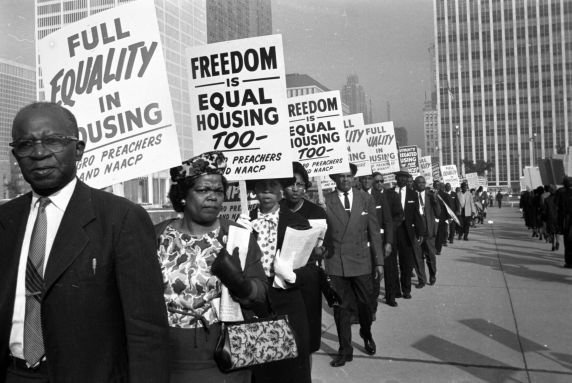This vintage black-and-white photograph depicts a solemn protest scene, likely from a past era. In the foreground, a line of African American men and women stand holding various signs, including messages like "Full Equality in Housing" and "Freedom is Equal Housing Too." The demonstrators are dressed formally, with the men in suits and ties, and the women in dresses, some carrying purses. The individuals' expressions are serious, many gazing directly at the camera, reflecting the gravity of their cause. The grey-toned ground and the multi-storey buildings in the background emphasize the urban setting of this powerful demonstration advocating for equal housing rights.